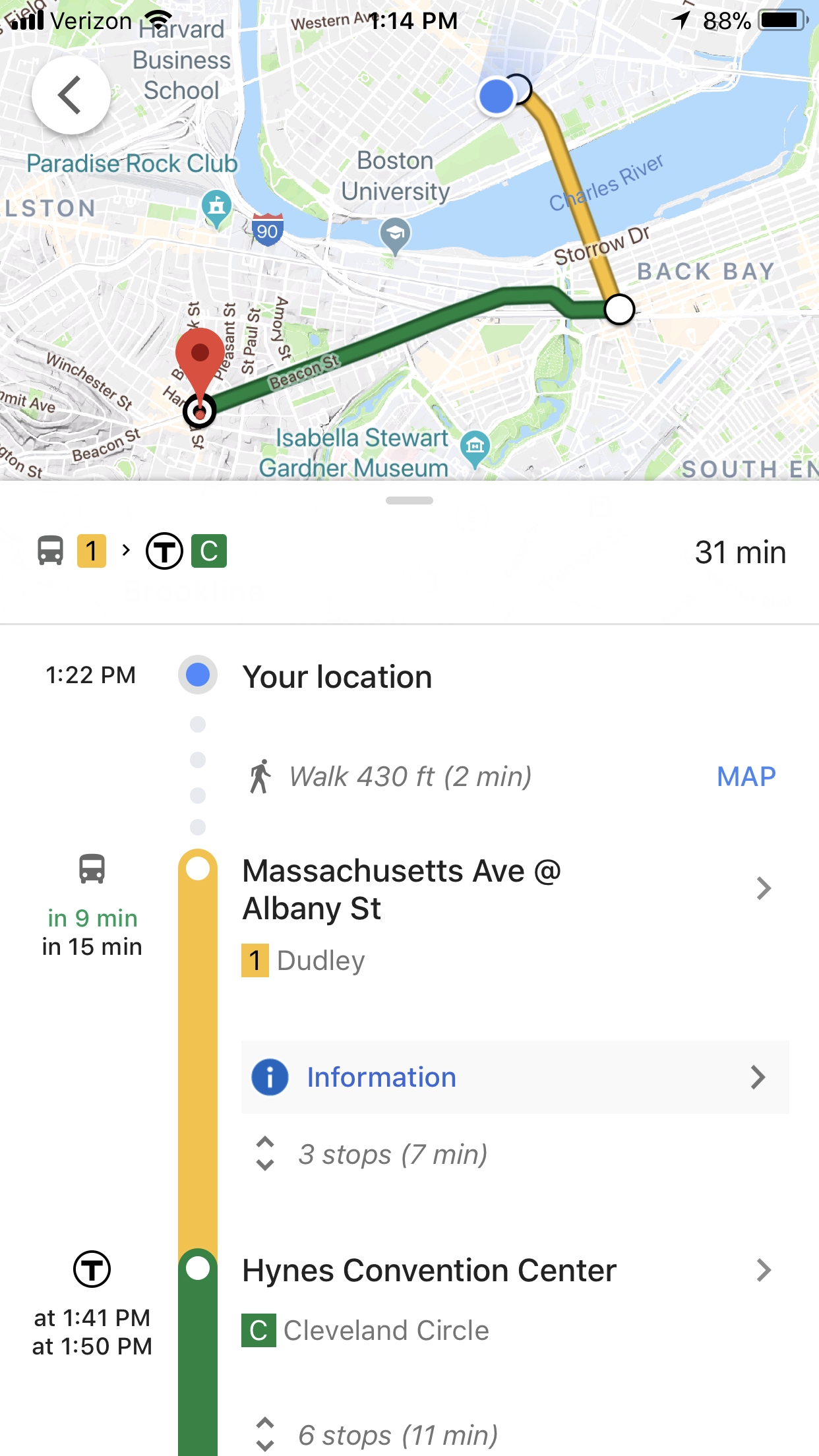The image displayed on a smartphone screen showcases a detailed navigation map around the Boston University area. The top-left corner displays signal indicators, while the center top shows the time as 1:14 PM. The battery indicator on the top right indicates 88% battery remaining. The map is superimposed with a planned route from one side of the Charles River, moving towards the Haynes Convention Centre. 

The route includes different modes of transportation: a 430-foot walking segment, followed by a bus journey starting from Massachusetts Avenue and Albany Street, and concluding with a taxi ride to the final destination. Each segment of the journey is meticulously detailed with the number of stops and estimated duration for each mode of transport. Additionally, the left-hand side provides information on typical travel times for these various transport options.